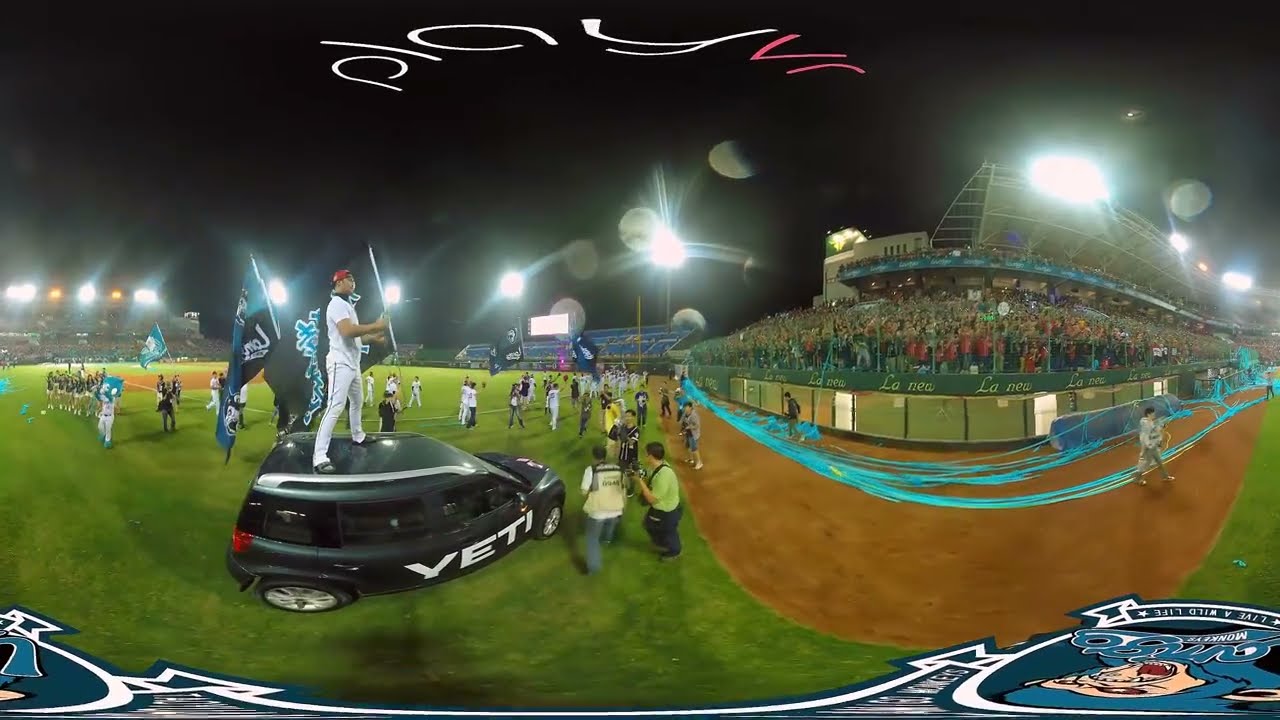The image is a detailed panoramic shot of a sports field set outdoors, under a dark sky illuminated by stadium lights, suggesting it's taken at night. The central focus is on a dark green SUV with the word "Yeti" in white letters on its side door. Positioned mid-left in the image, a man stands on top of the SUV, legs apart, facing the right, holding a black flag with blue letters. He is dressed in white clothing and wears a red baseball cap. 

Surrounding the vehicle, players and fans are visible; some players are holding blue flags that match the flag held by the man on the SUV. The field itself, which is mostly covered in grass with occasional dirt patches, is filled with spectators both on the field and in the stands. 

In the stands, a large number of fans can be seen, and along the front of the stands spans a teal blue material, possibly a net or banner, being managed by some individuals. On the far edges of the field, soil and dirt visually demarcate the transition to the stands filled with excited onlookers. An array of people in diverse uniforms—white, blue—and some casual photographers are visible throughout the scene.

At the top of the image, white and pink text reads "Play VR" overlaying the night sky. The bottom corners of the image feature distorted illustrations of what appears to be a mascot, contributing to the vibrant, bustling atmosphere of the event. The field, spectators, and activities emphasize the lively environment of this sporting event, likely set in a baseball park.